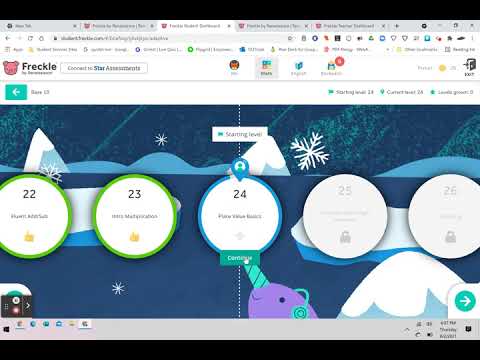In this image, we see an open browser window with five visible tabs. The focus is on the third tab, positioned in the middle. Although most of the text on this page is blurred, we can discern some figures and partial details. Notably, the image contains five circular icons. 

The first two circles are green and labeled with the numbers '22' and '23'. The '23' icon features a thumbs-up symbol. The third circle is blue, marked with the number '24', and appears to have the cursor hovering over it. The remaining two circles are greyed out or appear locked, indicating inaccessibility or incomplete status.

Additionally, at the bottom of the image, the taskbar is visible, displaying icons for various applications, including Google Chrome, Microsoft Edge, Email, and File Explorer.